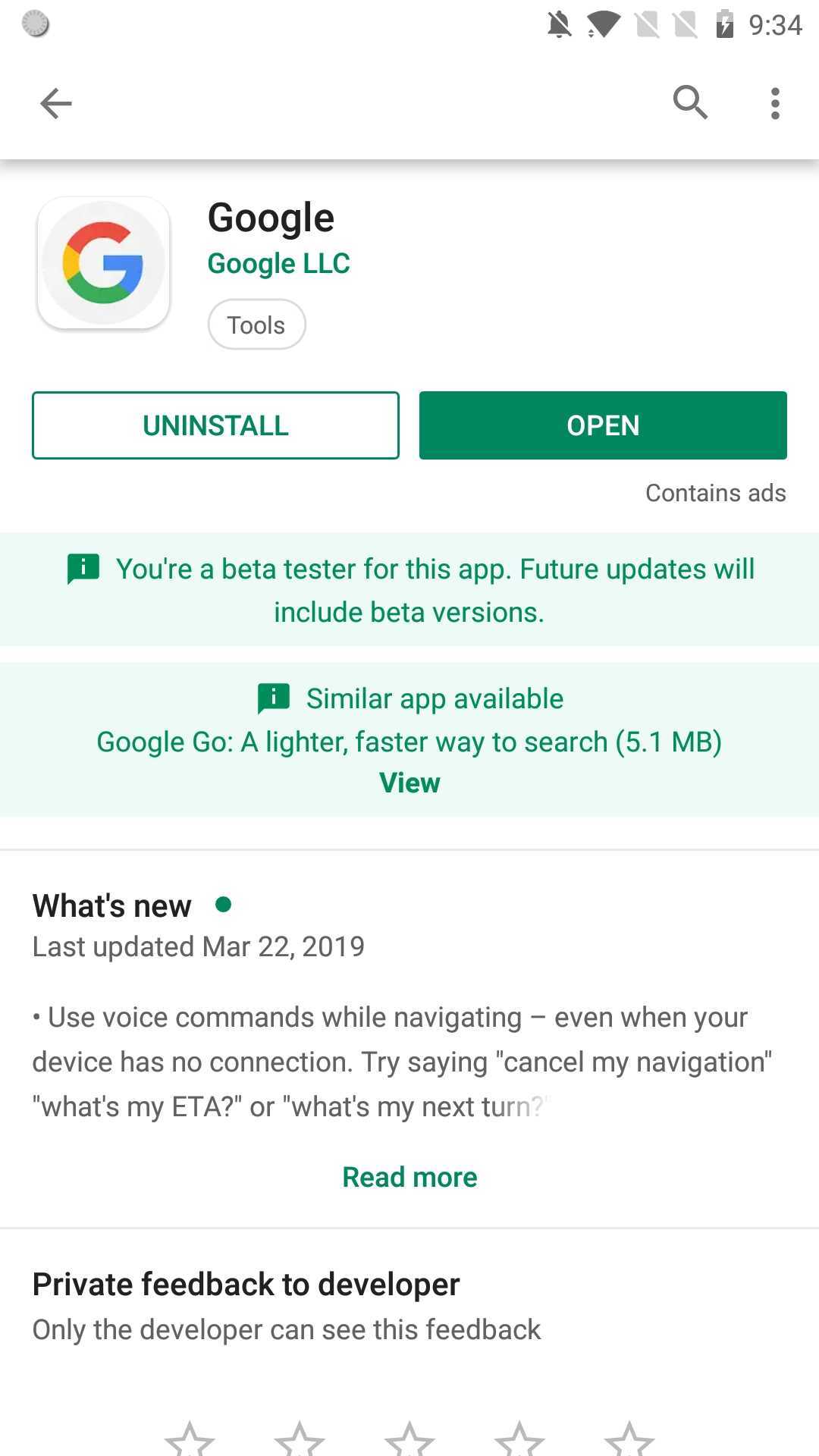This detailed caption describes a screenshot captured on an Android phone from the Google Play Store, specifically showcasing the Google app developed by Google LLC. The user has installed the beta tester version of this app. Alongside, the screenshot mentions similar apps like Google Go, a lighter and faster alternative that only occupies 5.1 MB of storage space. The user has clicked on the "Open" button, displayed in green, indicating that the app is already installed. Additionally, there's an option to uninstall the app. 

The rating section reveals that the user has not yet rated the app, as all five stars remain blank. The screenshot provides information about the current version of the app, which was last updated on March 22, 2019. This version includes features such as command words for navigation and an estimated time of arrival functionality. The layout of the page is predominantly white, with any information related to the beta tester version highlighted in light pastel green, accompanied by text in a forest green color.